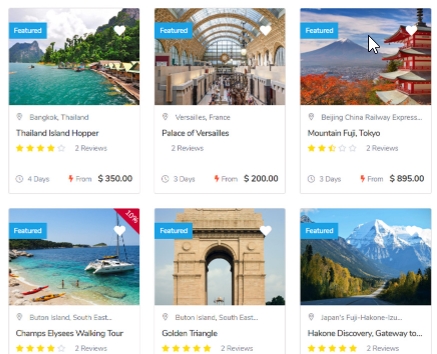The screenshot displays six potential travel destinations, each with various ratings and prices. 

1. **Thailand's Island Hopper**: This trip is rated 4 stars and costs $350.
2. **Palace of Versailles**: Listed at $200, with no star rating visible.
3. **Mount Fuji in Tokyo**: Rated 3 stars and priced at $8.95.
4. **Champs-Élysées Walking Tour**: Displays a review, with no specific star rating or price.
5. **The Golden Triangle**: Similar to the previous option, it only shows a review.
6. **Haozhong Discovery Gateway**: Holds a 5-star rating, possibly indicating a higher cost due to the challenging nature of the trip.

These options are accompanied by ratings and prices, providing a clear overview for potential travelers.